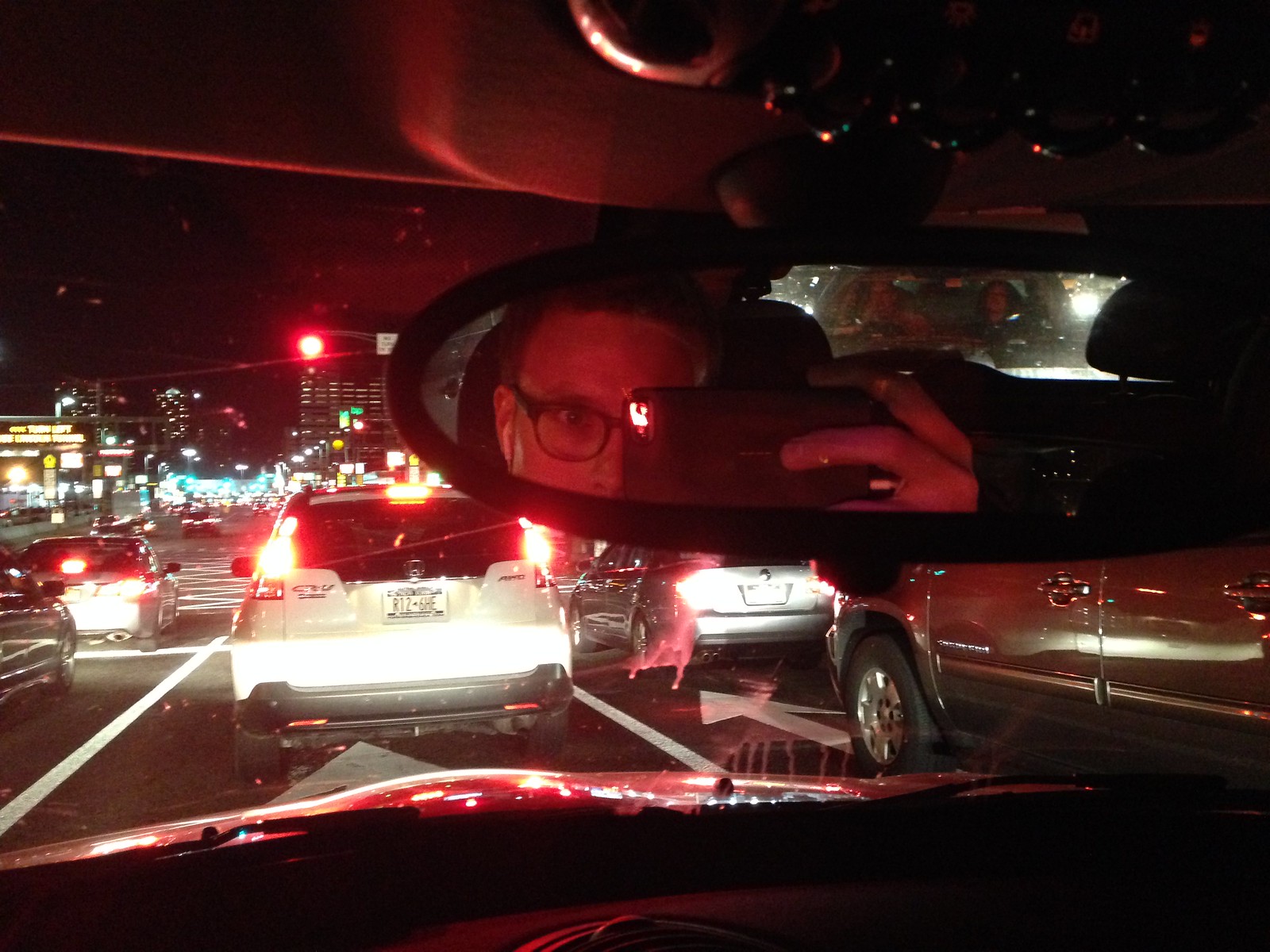The image captures the inside view of a car at night, looking outward through the front windshield. The rearview mirror in the photo reflects the photographer: a man with short brown hair wearing black glasses, holding a camera. Behind his car, another vehicle is visible, occupied by two individuals. The scene outside the windshield reveals a bustling city street, illuminated by numerous city lights and building illuminations. Immediately ahead, five cars are visible, and further in the distance, more vehicles can be seen. A traffic light, glowing red, is positioned two or three cars ahead. The photo effectively combines elements of the immediate car interior with the dynamic urban landscape beyond, encapsulating the vibrant nighttime atmosphere of the city.